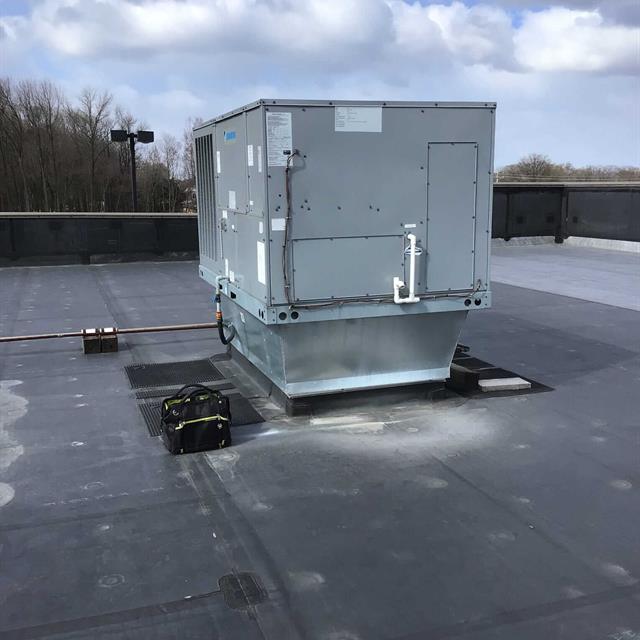The image depicts a rooftop scene viewed from above. The roof is predominantly gray with white specks and patches scattered across its surface. A mostly black bag with some distinguishing features lies on the roof. The blue sky is clear, indicating daytime, and although clouds are visible, it does not appear overcast or suggest imminent rain. Leafless trees and light posts provide perspective, appearing shorter in comparison to the vantage point of the roof. Black and brown cords wrap around parts of the rooftop, their purpose unclear. Additionally, vents are positioned on the left side of the roof.